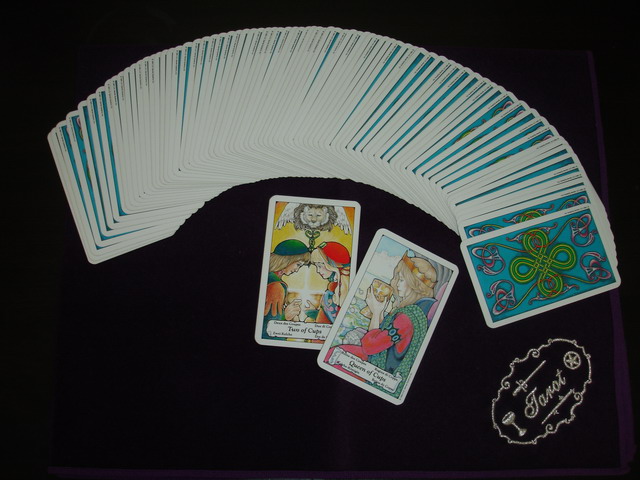The photograph showcases a fanned-out deck of tarot cards arranged in a U-shape, with two cards prominently displayed in the foreground. On the left is the **Two of Cups** card, depicting a blonde-haired man with a green hat and green shirt with orange sleeves, his forehead touching that of a blonde-haired woman wearing a red hat and a blue and red dress. Between them hovers a winged lion figure. The label "Two of Cups" is inscribed at the bottom of this card.

Adjacent to it, slightly overlapping, is the **Queen of Cups** card. Here, the same blonde-haired woman appears alone, drinking from a cup. She is dressed in a long red sleeved dress accentuated with a green tunic. The backs of the tarot cards feature an intricate design: a green, Gaelic, figure-eight-like pattern set against a sky blue background with a white border, interwoven with a detailed purple flower motif.

In the bottom right corner of the spread, a small patch bears the word "Tarot" in cursive. Surrounding it are the symbols of the four suits in the tarot deck: a sword above, a wand below, a pentacle to the right, and a cup to the left of the word, all enveloped in an ornate vine-like design. The entire arrangement rests on what appears to be a plush, velvet-like blanket or tablecloth, enhancing the mystical allure of the scene.